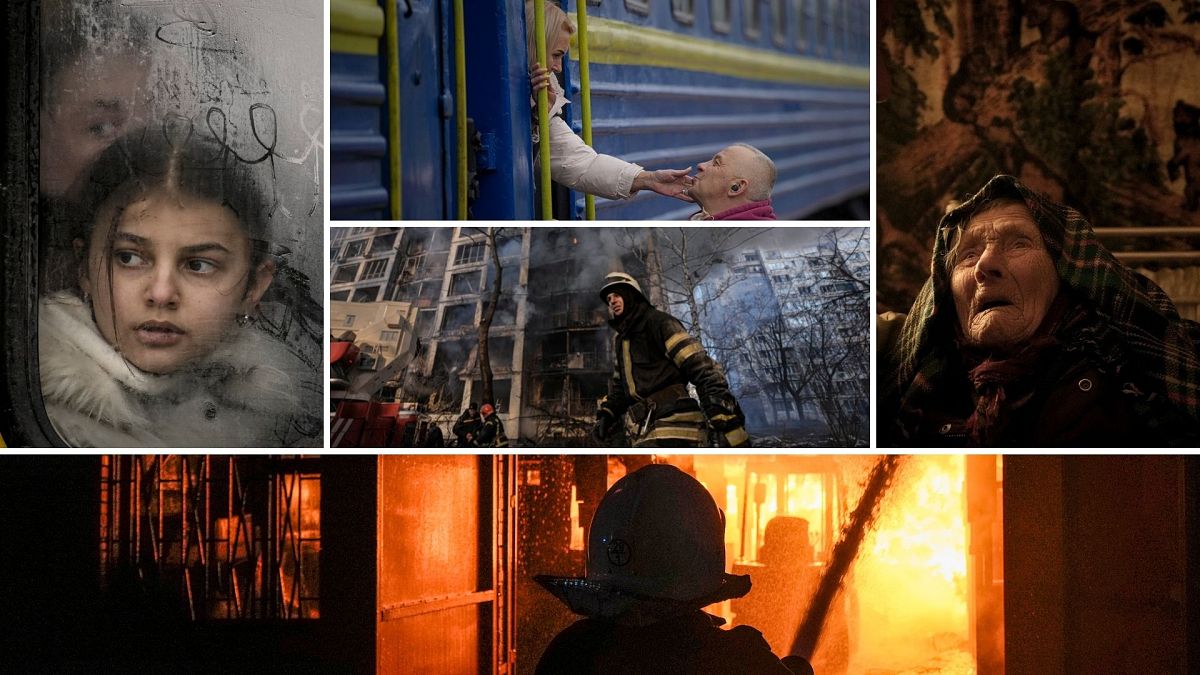The image is a composite of five distinct panels, each depicting various scenes of distress and resilience in a country undergoing turmoil. The largest panel stretches across the bottom and shows firefighters courageously battling a blaze inside a burning structure, the scene awash in an ominous orange glow. Above this, four smaller panels are arranged in a 2x2 layout. 

In the top left portrait panel, a young girl gazes pensively out of a frosted window, possibly from a bus, with the vague silhouette of a larger figure behind her, adding to the sense of uncertainty and foreboding. The central top panel captures a poignant moment as a woman extends her hand to touch the face of a kneeling man, seemingly bidding farewell, against the backdrop of a blue and yellow train. Directly below this, a firefighter is depicted in front of a smoking building, amidst high-rise structures, possibly running toward the firetruck in the background.

The top right portrait panel features an old woman with a sorrowful expression, looking into the distance as if seeking solace. She is adorned with a headscarf and stands before a mural-like backdrop. Each panel encapsulates themes of human emotion, bravery, and the stark realities faced during catastrophic events.